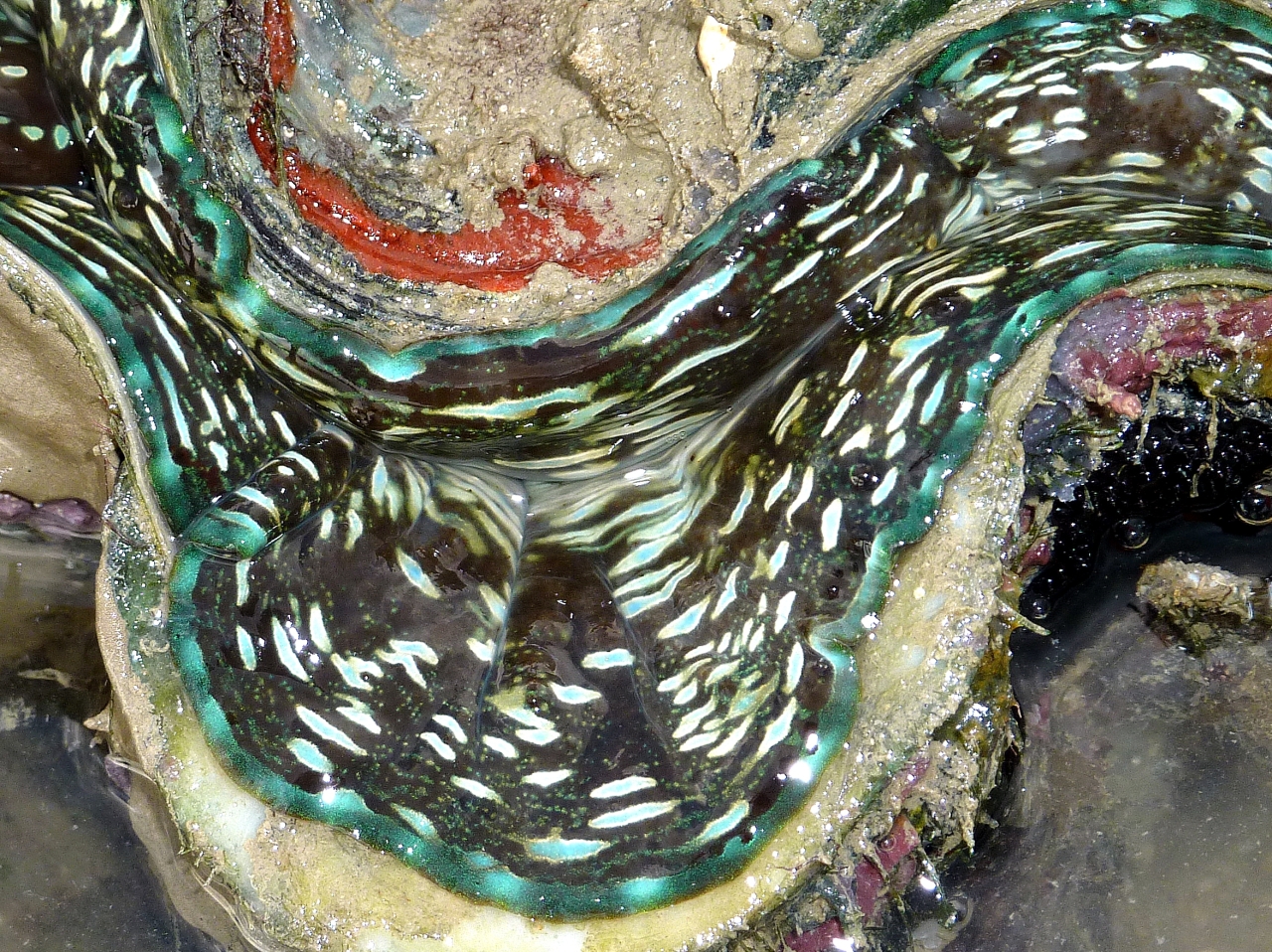In this detailed landscape-oriented color photograph, the subject features an intricate and abstract pattern created by swirls of colored glass, giving the image a striking and confusing appearance. At the center lies a half-circle shape with a streak of red near its base, suggesting intense contrast. Surrounding it is a dark, swirling design accented by elliptical white dots and splotches of rich green hues. These elements resemble the wavy ridges of a shell, possibly reminiscent of a giant clam's mouth. Below this pattern, the glass transitions into representations of what appears to be a moist, freshly dug brown mud accentuated by an orange blob, adding to the visual complexity. The overall composition is marked by the interplay of a dark background, evocative of a shell’s gray coloration, and aqua-colored rims seen from above, accompanied by subtle crystallized textures with spiky formations and a creamy edge. The corners of the image are framed by gray rocks, implicitly grounding the abstract swirls in a realistic, almost photographic representation.